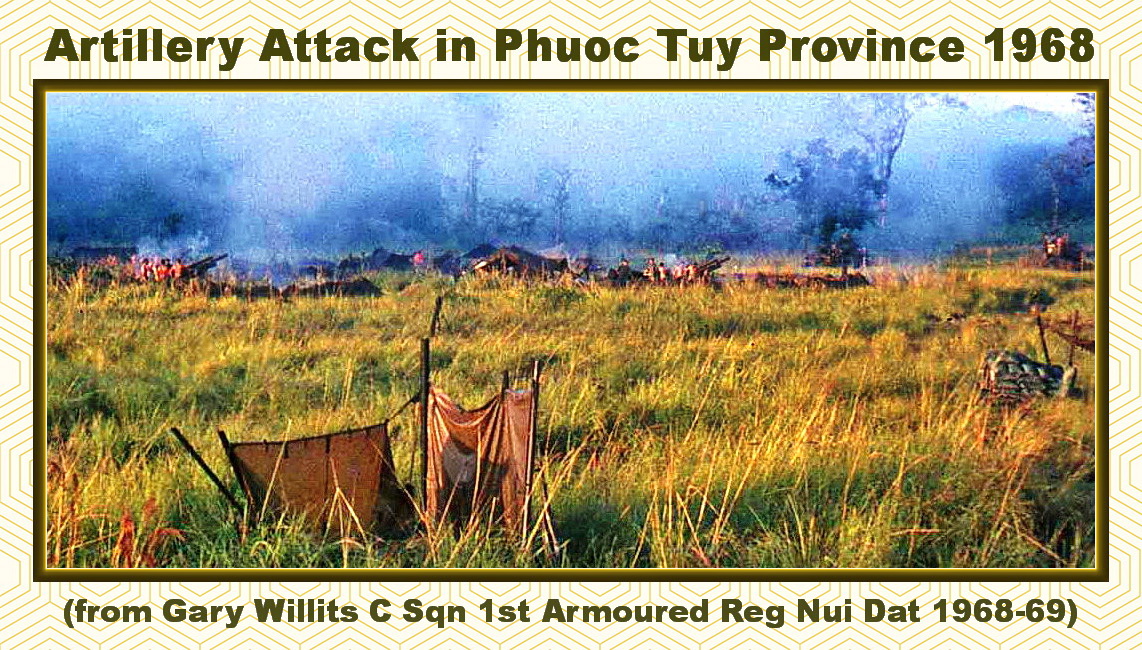The image, which appears to be a painting or an illustration, is bordered and depicts the aftermath of an artillery attack in Phước Tuy Province, 1968. At the top of the border, inscribed in large green font, are the words "Artillery Attack in Phước Tuy Province, 1968," while the bottom border reads, in smaller green font, "from Gary Willett, C. SQN 1st Armored Regt, Nui Dat 1968-69."

The scene within the borders presents a grassy landscape in the foreground, interspersed with light green, yellow, and greenish blades. A partially collapsed orange tent lies prominent in the foreground, suggesting recent disturbance or destruction. In the mid-ground, a thick plume of white smoke rises from the grass, indicating recent artillery fire. The background is dominated by an indistinct tree line, slightly blurred by a mix of mist and smoke. There are hints of additional tents and figures, possibly soldiers, though these details are blurred and difficult to discern due to the painterly style of the image. The sky above transitions from light blue to white, adding to the overall haziness of the scene.